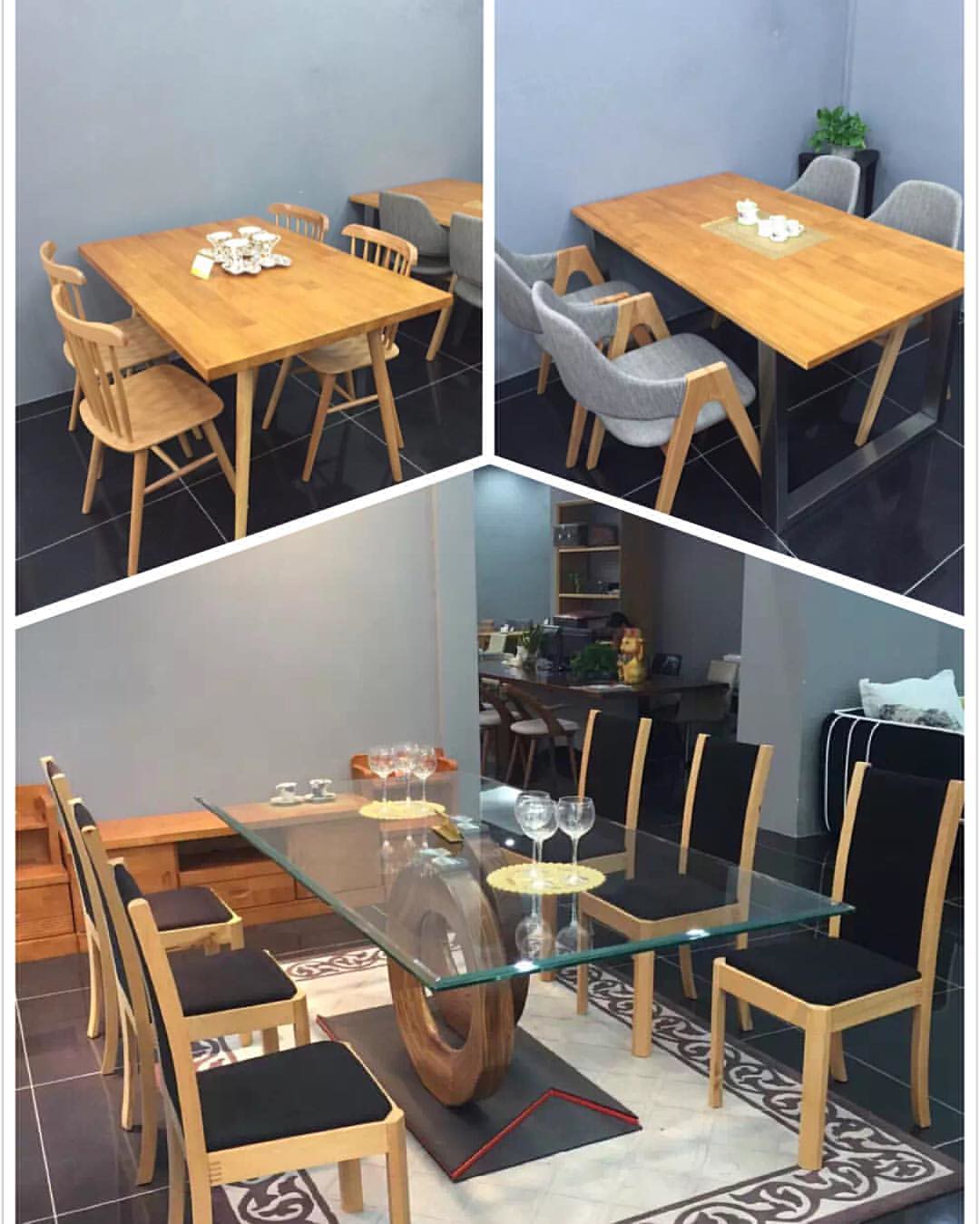The image is a detailed color photograph designed as an illustration, likely for an editorial or publication, split into three distinct sections resembling a peace sign. The bottom section, shaped like a roof and approximately twice the size of the upper sections, features a sophisticated dining table with a long, elegant glass tabletop supported by two large, centerless wooden rings. Surrounding this table are six wooden-framed chairs adorned with black cushions and backs, complemented by glassware on the table. The top left section showcases a simple, light wooden dining table with round legs, accompanied by four matching wooden chairs with dowel backs, suggesting a casual, restaurant-like ambiance. The top right section presents a modern wooden tabletop with contrasting black metal beams for legs, paired with advanced gray-felt chairs that have wooden legs and armrests. The entire collage is characterized by a harmonious blend of grays, browns, and light blues, with white borders delineating the distinct table settings.